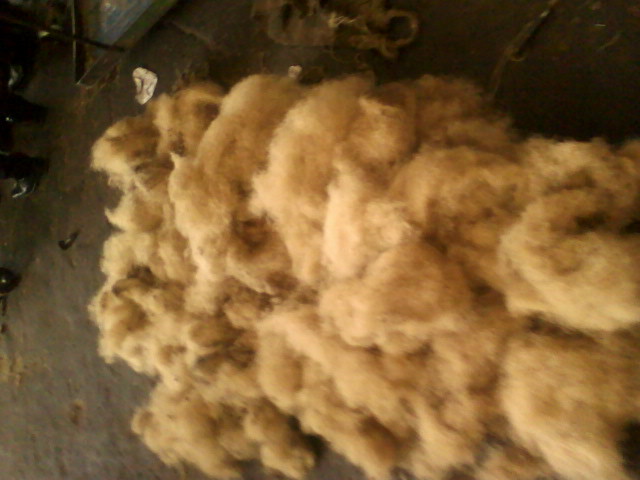This is a sideways, dark, and grainy photograph that appears aged and slightly torn in spots. The image predominantly features a large, light brown fur spread across the ground, likely from a sheared animal, resembling sheep fur. In the foreground, the fur appears very blurry, while in the background, it transitions to a darker brown shade. The ground beneath the fur and surrounding area is dirty, with dark brown and gray hues, suggesting a frequently used space.

In the background on the left side of the photograph (or the top edge, due to the sideways orientation), there is a pair of black dress shoes pointing away from the viewer, indicating the presence of a person. Additionally, a gray tray, possibly part of a shelf, is visible in the top left corner. The overall scene gives a chaotic impression of an animal shearing area, emphasized by the dark tones and grainy quality of the photograph.